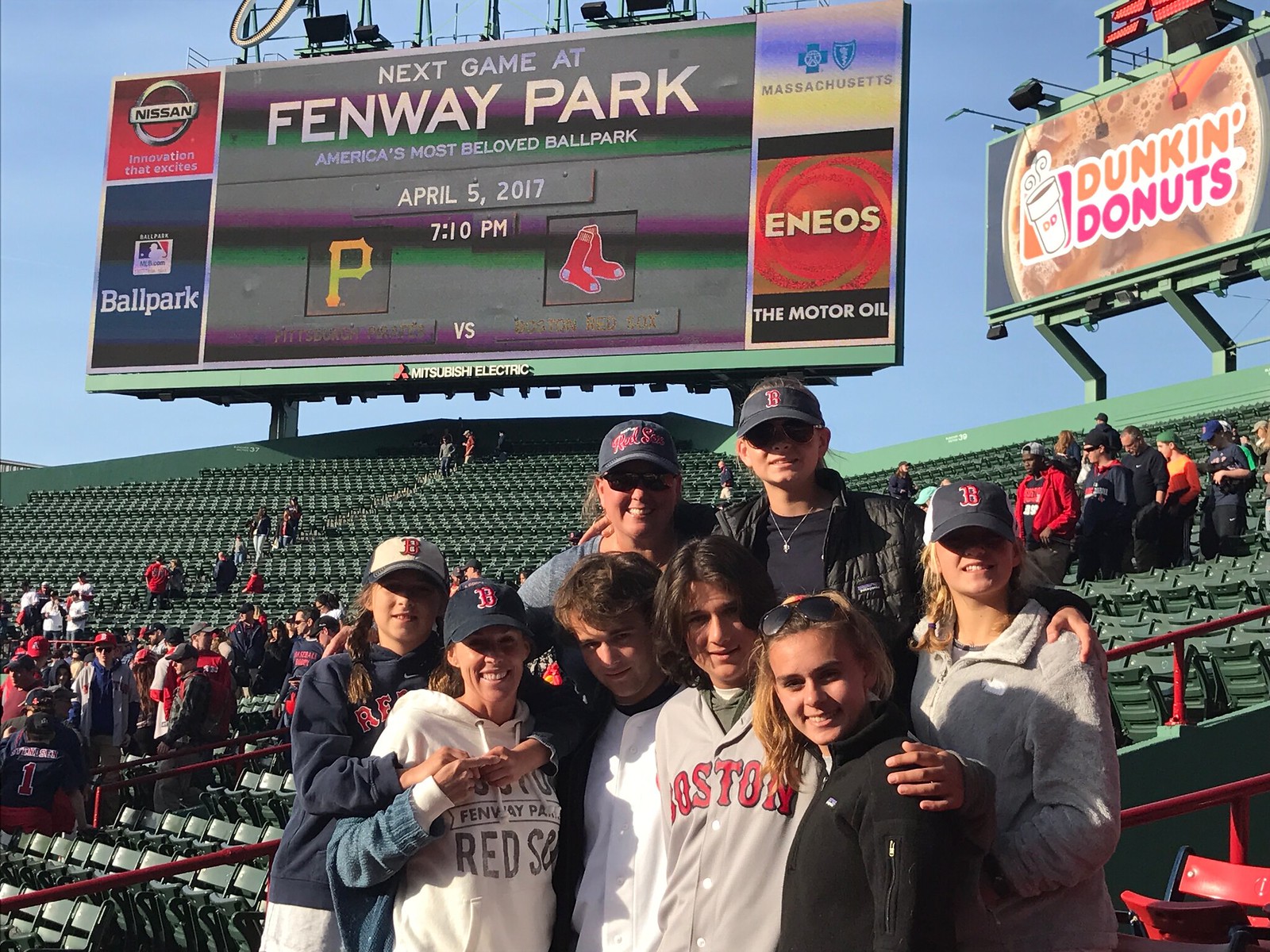A happy family of eight, consisting of two adults and six children, is captured enjoying their day at Fenway Park, home of the Boston Red Sox. They are standing in the mostly empty outfield bleachers, which are painted green, with arms wrapped around each other, beaming at the camera. The background prominently features a large scoreboard displaying "Fenway Park" and an announcement for the next game: the Pittsburgh Pirates vs. the Boston Red Sox. To the right of the scoreboard is a notable Dunkin' Donuts sign, among other advertisements like Nissan, Blue Cross Blue Shield of Massachusetts, Major League Baseball, and Ineos Motor Oil. The beautiful, clear blue sky without a cloud in sight suggests it's a delightful mid-afternoon, making it a perfect day for a memorable family outing.